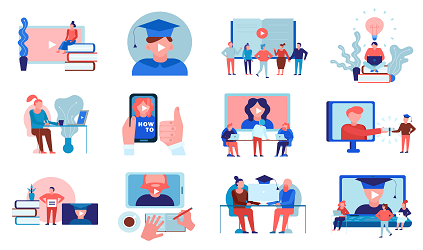The image is a composite of twelve minimalistic digital artworks arranged in three rows of four columns, each with themes predominantly in red, white, and blue hues. The scenes depicted are rendered in a clip-art style with nondescript, faceless characters featuring only basic details like hair and ears. Many of the images have play buttons, suggesting the presence of videos.

In the top left corner, a character sits on a stack of books with a pink board and an arrow pointing right behind them. Next, a graduate wearing a blue cap, their face obscured by a play button, stands with a blue circle backdrop. Adjacent to this, an open book is displayed with people milling around. The final image on this row shows a person with a lightbulb overhead, symbolizing an idea or moment of inspiration.

The middle row starts with a person seated at a desk with a computer, followed by a phone with someone giving a thumbs up. The third image displays a large screen TV with a person standing in front of it, and another image features someone handing an item to another person, possibly at a desk.

The bottom row includes a figure beside a screen and an open book. Next to it, an image of a phone shows a scene with a play button, hands writing in a book, and a coffee cup nearby. The next image depicts two people at a table with graduation caps, while the final scene features a large screen showing a graduate in a cap with people standing before it.

Overall, the artwork emphasizes educational and technological themes with frequent imagery of graduates, books, computers, and play buttons indicating multimedia content.